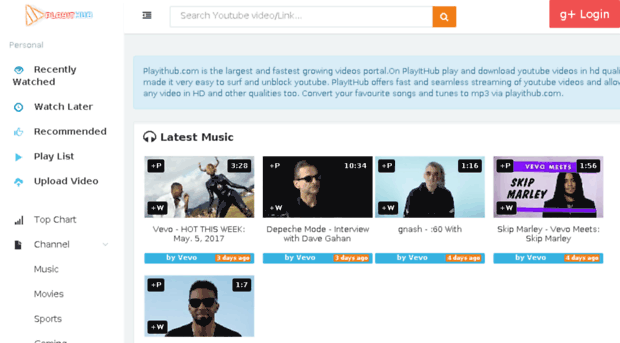This cropped screenshot features the PlayItHub website as viewed on a desktop. The background is predominantly white, with the PlayItHub logo positioned in the top-left corner. Running vertically down the left side of the page are various navigation categories. Starting from the top, there is a small gray label that reads "Personal". Immediately underneath, you'll find categories labeled in larger text: Recently Watched, Watch Later, Recommended, Playlist, and Upload Videos.

Further down, another set of categories is listed vertically in smaller gray font: Top Chart, Channel, Music, Movies, and Sports, continuing off the visible section.

On the right side of the screenshot, the background shifts to gray. Dominating the top-center of this section is a prominent blue banner which reads, "PlayItHub.com is the largest and fastest growing videos portal on PlayItHub. On PlayItHub, play and download YouTube videos in HD," although the text is cut off.

Below this banner, there is a large white box. In the top-left corner of this box, it is labeled "Latest Music". Beneath this heading, a series of artist thumbnails are displayed horizontally, providing visual previews of music content available on the platform.